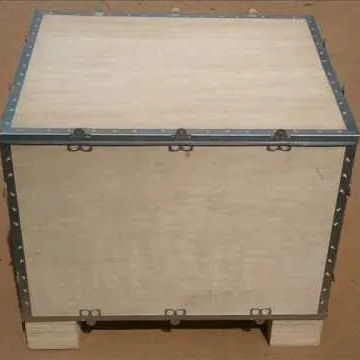The image portrays a small, rectangular wooden chest with dark gray metal framing along all the corners and edges. The wood has a textured appearance and is light brown in color, reminiscent of a material like balsa, though not likely balsa due to its typical use. The chest features three metal clips on the visible sides and hinges, suggesting the presence of a lid. It rests on four block-like wooden legs, which appear to be offcuts of 2x4 lumber, giving it a makeshift, unfinished look. The background is a plain light brown, possibly indicating a garage or workshop floor. The image is captured from a slightly elevated angle, offering a perspective from above and to the side, showcasing the chest's simple, functional design amidst its utilitarian backdrop.